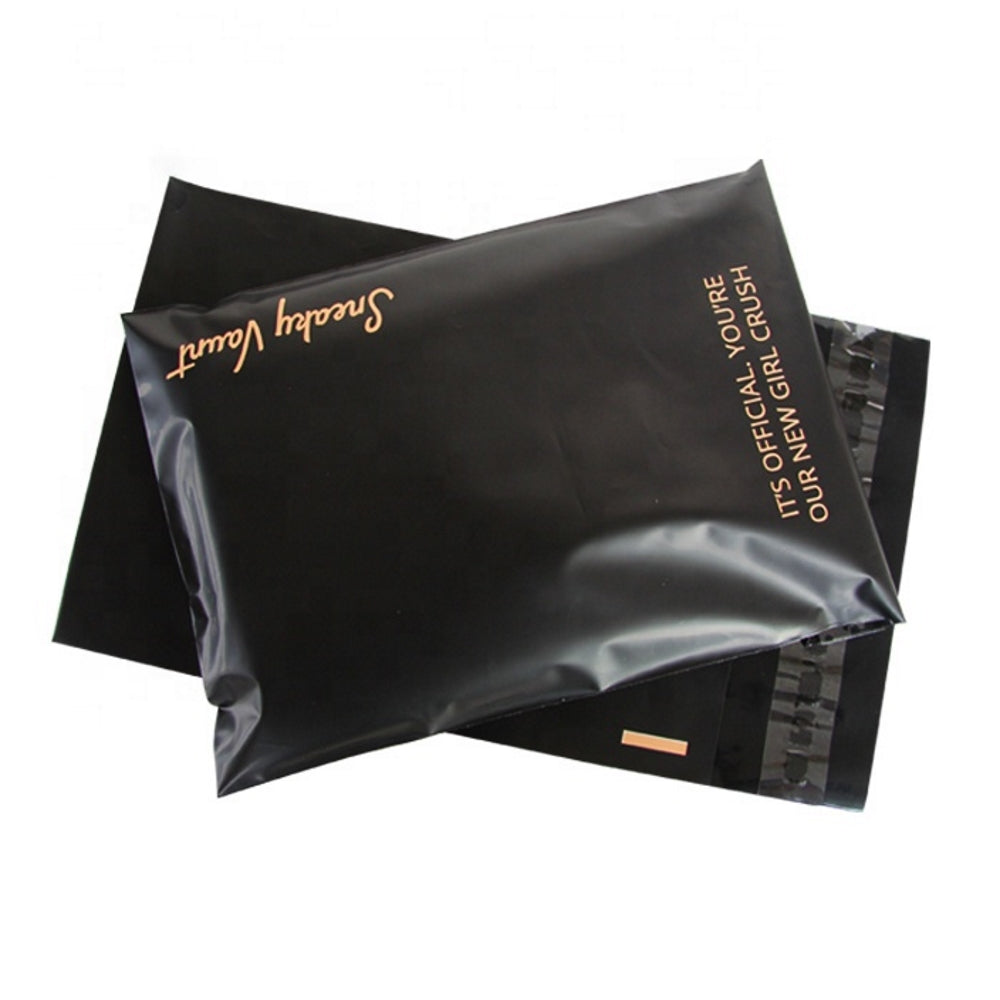The image features a completely white background, which starkly contrasts with two black plastic pouches centered in the frame. The bottom pouch appears flat and has a clear strip indicating it can be filled and sealed; it tilts slightly downwards to the right. The second pouch, placed above the first but tilting to the left, looks like it already contains something. Notably, the packaging displays faint salmon-colored text. In the upper right corner, an upside-down cursive script reads "Sneaky Vaunt," presumably the company name. Along the right side of the pouch, the tagline says, "It's official, you're our new girl crush." This thoughtful design hints at the company's possible focus on discreet shipping, likely for sensitive or adult-themed products, providing their customers with privacy and a sense of excitement.